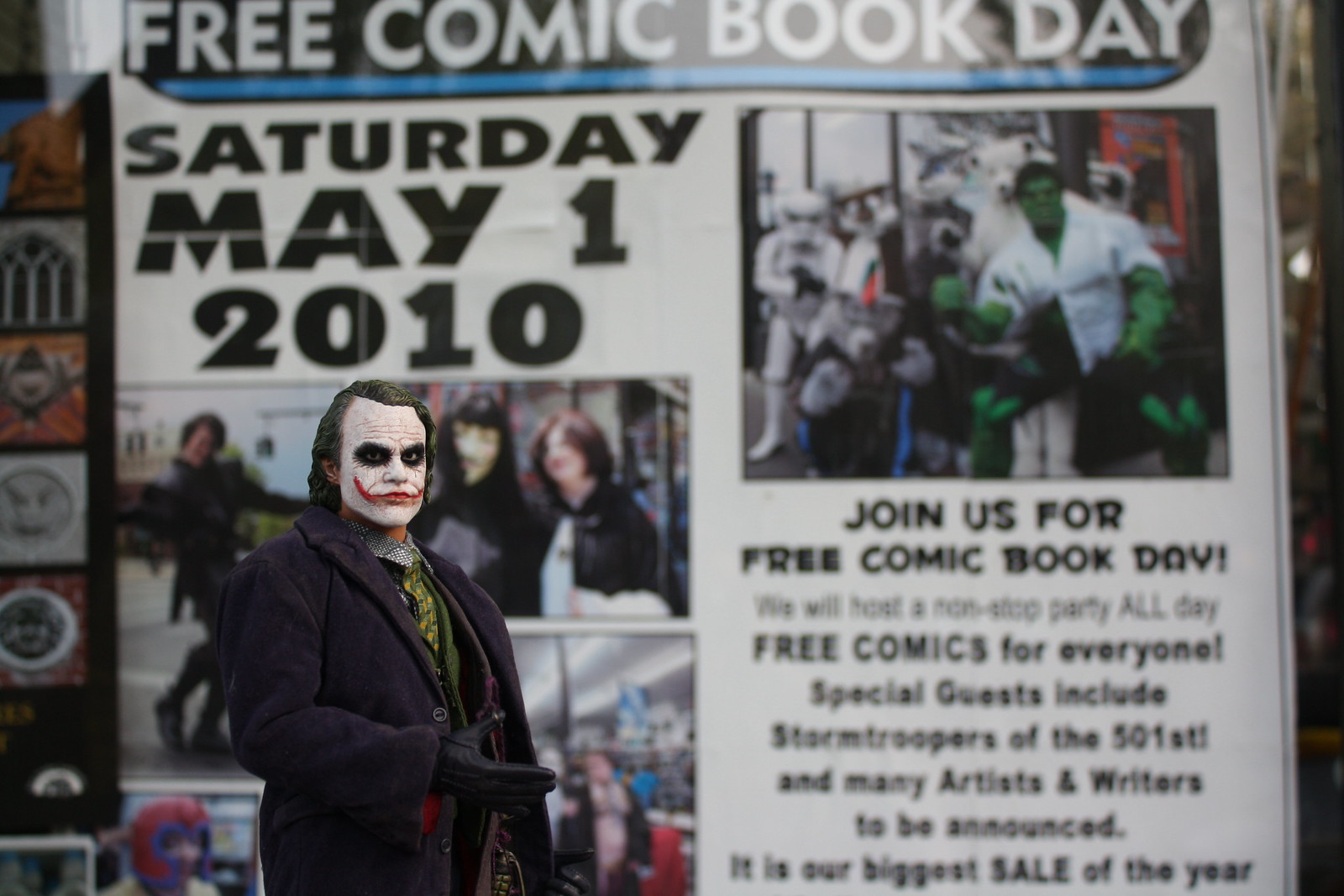In the foreground, a man is dressed as the Joker, reminiscent of Heath Ledger's portrayal, with meticulous details such as white face paint, an exaggerated red smile that curls upward on both sides, black circles around his eyes, and disheveled black hair. His costume includes a long black coat, black gloves, and a green vest. The coat is open, revealing more of his attire. Behind him, a poster advertises "Free Comic Book Day" scheduled for Saturday, May 1st, 2010. This promotional sign, set against a white background, features images of iconic characters, including the Hulk on the right side and several cosplayers, some in black outfits, on the left. The text on the poster reads, "Join us for a free comic book day. Free comics for everyone. Special guests include Stormtroopers of the 501st and many artists and writers to be announced. It is our biggest sale of the year." The overall setting suggests the poster is part of a larger event, possibly a comic-con, where the Joker impersonator is participating.